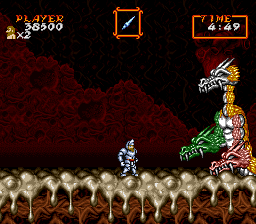A vibrant, digitized image reminiscent of a classic video game showcases an epic confrontation. Dominating the scene is a colossal dragon, its face gleaming silver with a striking contrast to its yellow neck and head. Uniquely, the dragon's limbs aren't typical appendages; its right arm takes the form of a green dragon head, while its left arm features the menacing visage of a red dragon. Opposite this formidable creature stands a diminutive knight, clad in shining armor, poised for battle on a rugged terrain that appears to be molten lava. The game interface is visible, with "Player" and a score of "38,500" displayed in the upper left corner, along with a small avatar and "x2" symbol. In the top right corner, a timer reads "4:49". The entire scene is encompassed within a black square, evoking nostalgia for vintage gaming aesthetics.